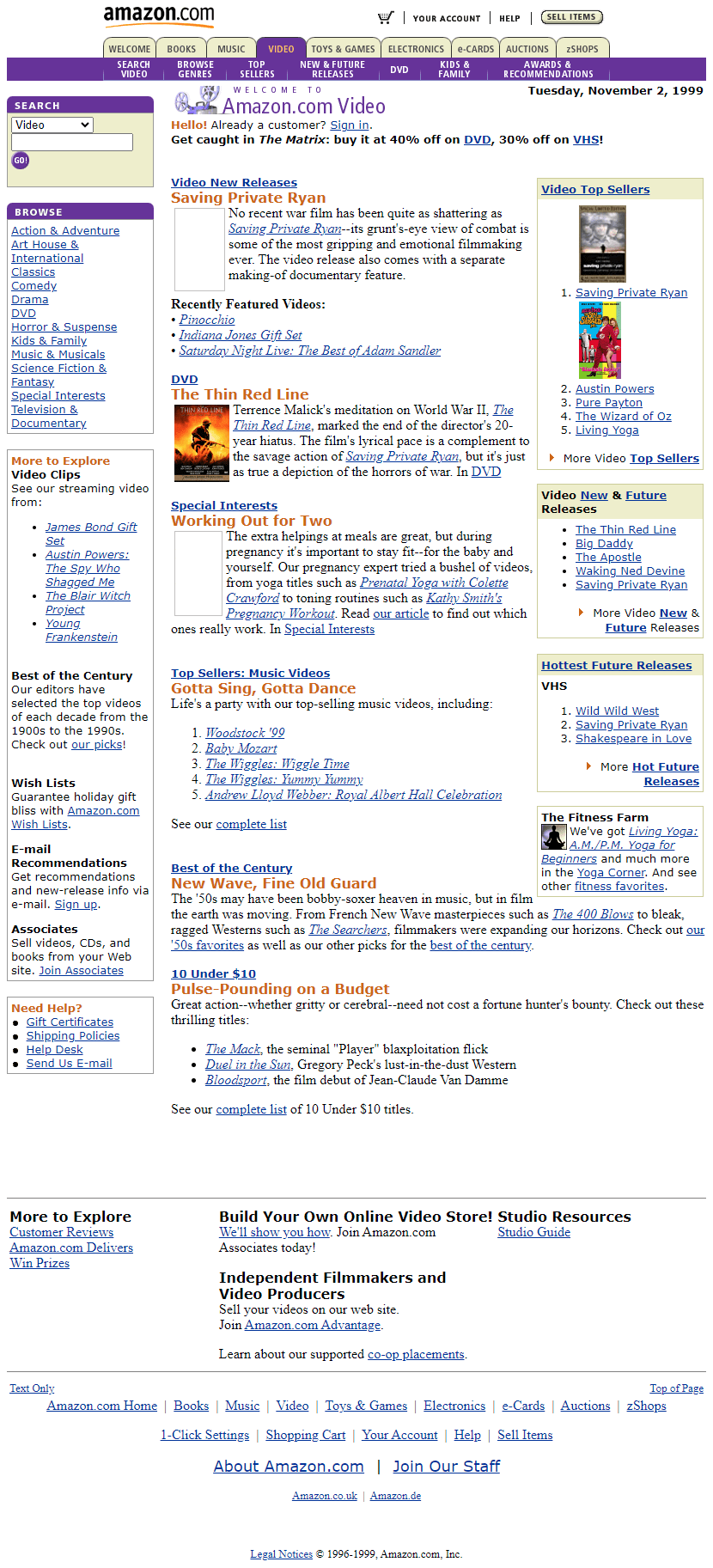The image appears to be a screenshot taken from the Amazon.com website, specifically from the Amazon Video section. The logo for Amazon.com is present but the image quality is too poor for detailed legibility of the elements. The visible text includes phrases such as "Amazon Video," "Saving Private Ryan," and "The Thin Red Line." A drop-down menu labeled "Video" is visible, along with a text box inside a gray rectangle bordered in dark blue at the top.

Below this section, there is a cluster of blue hyperlinks interspersed with red and black text. These hyperlinks seem to be organized with either hyphens or bullet points next to them. On the right side of the image, several thumbnails are visible. One prominent thumbnail features black, yellow, and orange colors, located underneath the mention of "The Thin Red Line." Even smaller thumbnails are present on the far right, each accompanied by blue hyperlinks beneath them. Additional clickable options are located at the bottom of the image, but the blur makes it difficult to decipher the specific content or text in these areas.